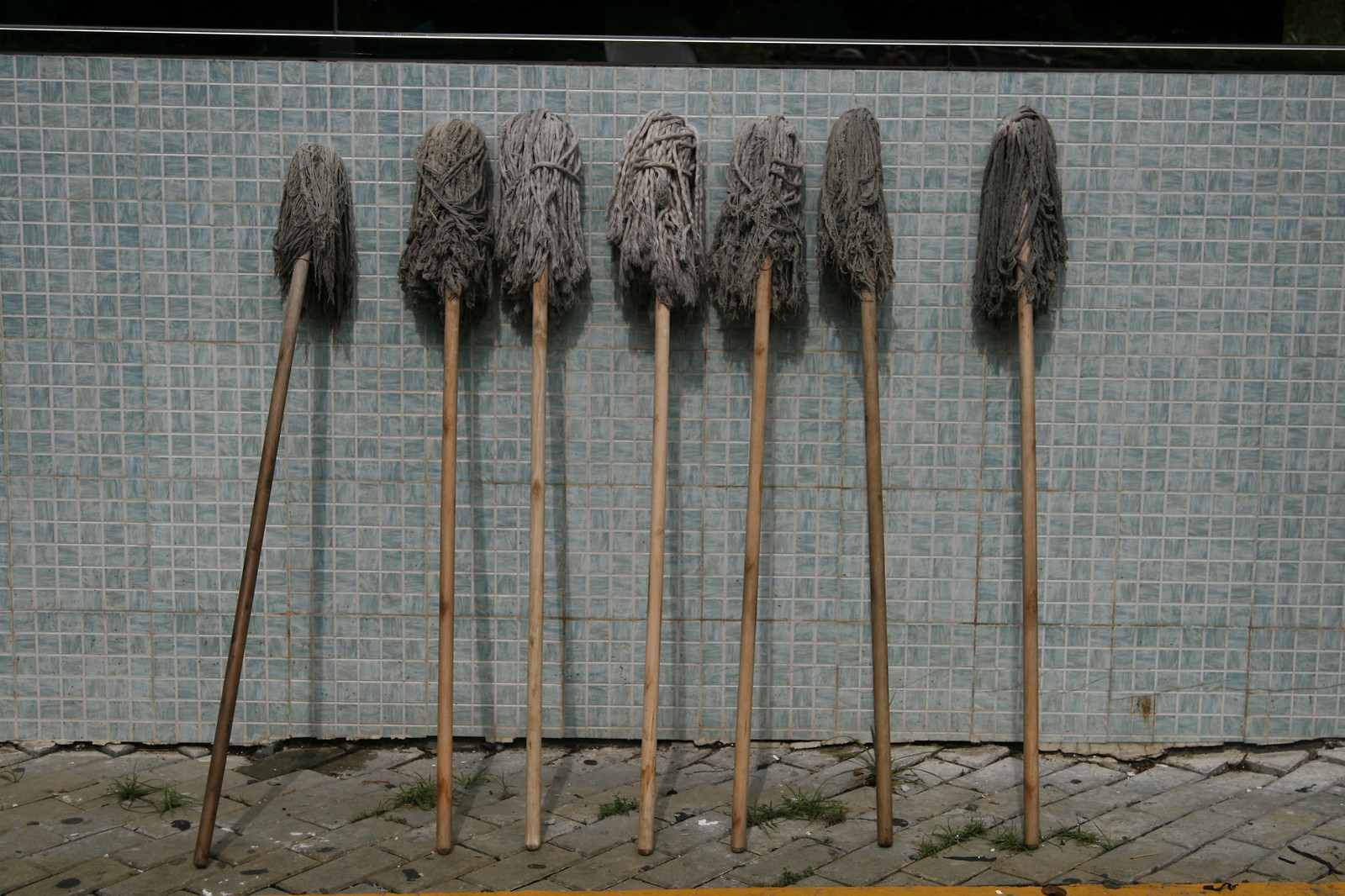This photograph features seven well-worn mops leaning against a wall adorned with intricate light blue and white tile patterns. The tiles are small squares grouped into larger squares, interspersed with gray grout, and a dark strip runs along the top edge of the image. Each mop stands propped at a diagonal angle, with their wooden handles resting on a ground of old, grayish-brown brick paving. The mop heads, varying in shades of gray from light to dark, display signs of heavy use and dirtiness. The bottom edges of the mop handles are stationed less than a foot from the tiled wall. The overall composition includes minimal floor space, enhancing the focus on the repetitive, yet distinctively battered appearance of the leaning mops.